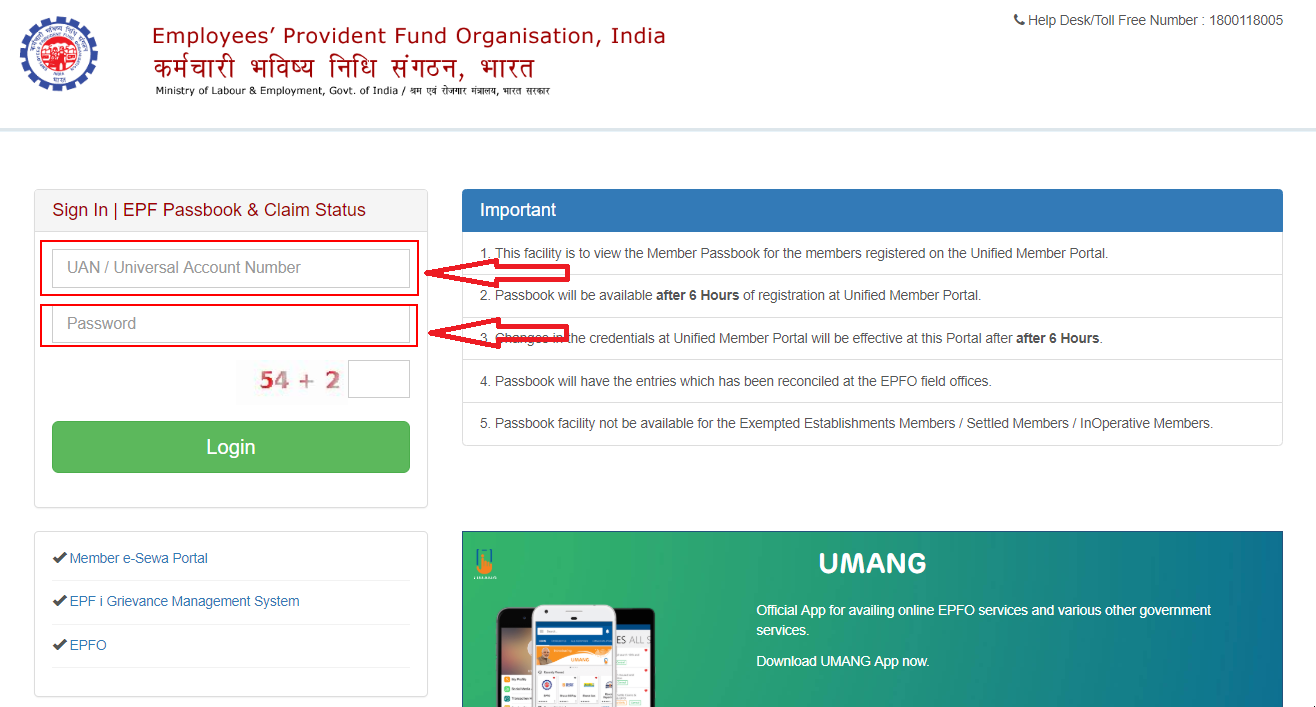This image is a screenshot from the official portal of the Ministry of Labor and Employment, Government of India, featuring the Employees Provident Fund Organization (EPFO). The background is predominantly white. In the upper left-hand corner, there is the EPFO logo, which includes a red, white, and blue circular design, accompanied by the text "Employees Provident Fund Organization India" in red ink. Beneath this, in small blue print, it reads "Ministry of Labor and Employment, Government of India."

A thin gray ribbon runs horizontally across the page, demarcating different sections. Below this ribbon, on the left side, there is a vertical column dedicated to user login information. At the top of this column is a light gray banner with the text "Sign In, EPF, Passbook, and Claim Status." Following this, there are input fields for the "UAN / Universal Account Number" and "Password," both outlined in red. Below these fields, there is a CAPTCHA featuring the equation "54 + 2" with a box to enter the answer, followed by a green "Log In" button.

Underneath the login section, there is a list of three options in bright blue with checkmarks next to each: "Member e-Sewa Portal," "EPF Grievance Management System," and "EPFO."

To the right of the login section, occupying the majority of the page, there is a prominent bright blue banner with the word "Important" written in white. Below this banner, five important points are listed. Additionally, there are two red arrows pointing directly to the Universal Account Number box and the Password box, emphasizing where users need to input their credentials.